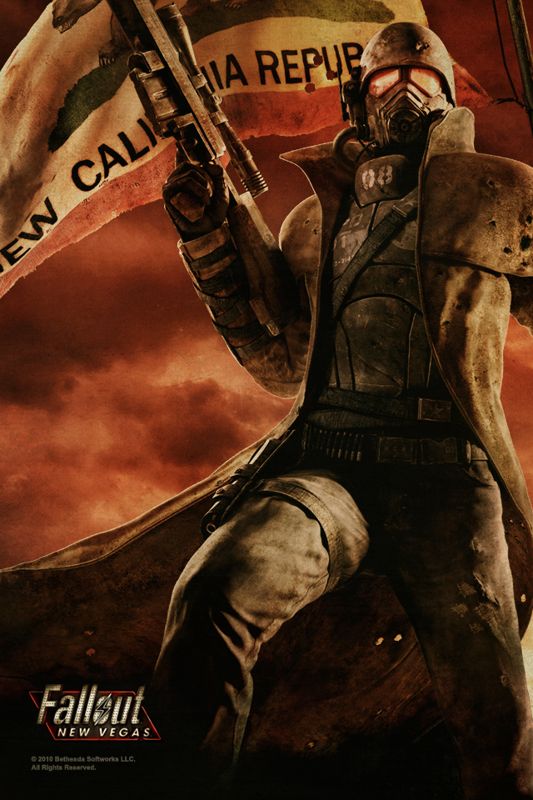The image is an advertising poster for the 2010 game Fallout: New Vegas by Bethesda Softworks LLC. It prominently features an NCR soldier standing in a dramatic pose. The soldier is clad in a detailed battle uniform that includes a grayish-brown leather jacket, a helmet with a gas mask and visor, and a long, western-style cape. He's holding a scoped sniper rifle pointed upwards. The soldier's attire is completed with some kind of body armor and a belt of bullets around his waist. In the background, a red and almond pink sky sets an intense scene, and the New California Republic flag, emblazoned with a bear, is clearly visible. The Fallout: New Vegas logo is situated in the bottom left corner, along with the copyright details stating "2010 Bethesda Softworks LLC, All rights reserved."